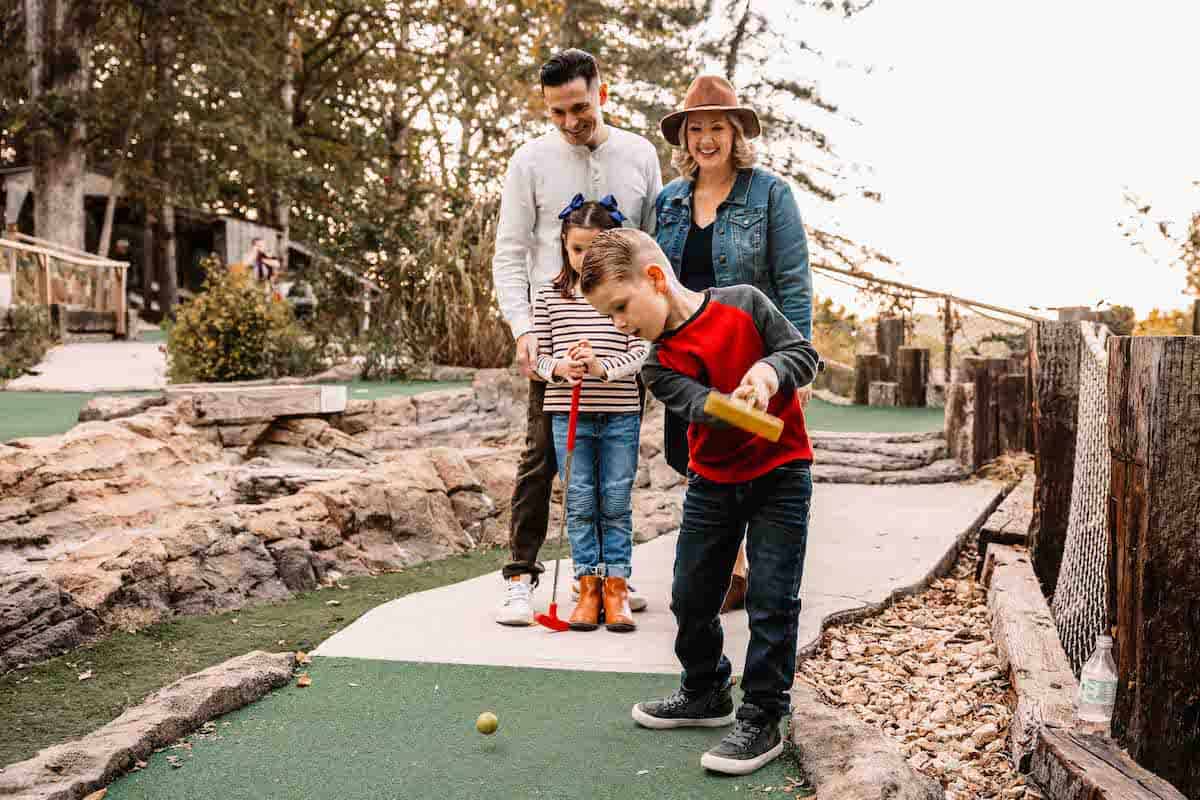In this realistic, horizontally-oriented photograph, a family of four—a mom, a dad, and their two children—are engaged in a game of mini golf outdoors amongst a natural-themed course featuring rocks, trees, and thick grass. The father, a white male in his 30s with black hair, is adorned in a white button-up shirt. The mother, also in her 30s and white, has blonde hair and is wearing a brown hat, a denim jacket, and a black shirt. Their daughter, approximately eight years old, is dressed in blue jeans and brown boots, paired with a white and black shirt. She is watching attentively alongside her mother and father. The son, who appears to be the girl's twin, is in mid-swing, having just hit a yellow golf ball with his yellow club. He sports black jeans and a red shirt. Additional details include a nearby mini-shed or cabin-type building to the left and a plastic bottle resting on a wooden board to the right. The atmosphere of the mini golf course is accentuated by the surrounding pine trees and manicured landscape, all bathed in bright daylight.